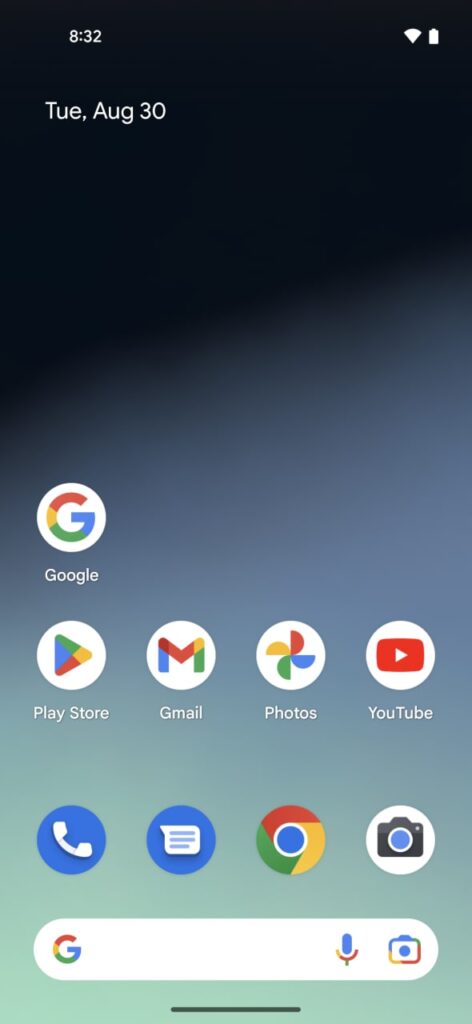The image displays a smartphone interface with a prominent background featuring a gradient. The gradient starts with an extremely dark navy blue at the top, transitioning smoothly to lighter blue shades, then to an aqua or teal blue, and finally morphing into a greenish hue at the bottom. The interface is active at 8:32 AM on Tuesday, August 30th, with fully charged battery and strong Wi-Fi signal indicators visible.

Central to the screen is the iconic Google logo, a stylized "G" with red, blue, yellow, and green segments encased in a white circle, accompanied by the text "Google" below it. Adjacent to this are several app icons: 
- The Google Play Store icon, featuring a right-pointing white triangle with colored segments (yellow at the tip, blue on the left, green on top, and red on the bottom).
- The Gmail icon, displaying a multi-colored "M" within a circle, incorporating blue, red, yellow, green, and orange.
- The Photos app icon, characterized by a multi-colored pinwheel formation with yellow, red, blue, and green hues.
- The YouTube icon, consisting of a red rectangular play button with a white arrow inside a white circle.

At the bottom of the screen is the dock, showcasing four essential application icons: 
- A green phone symbol for calling.
- A white text-messaging icon on a blue background.
- Another Google logo within a multicolored circle. 
- A camera icon.

Beneath these icons lies a transparent search bar with the Google "G" on the left and a blue and yellow microphone icon for voice search on the right. This bar also includes a camera icon, presumably for visual search functionality. There is a thin black line stretching across the middle of this search bar, adding a touch of separation.